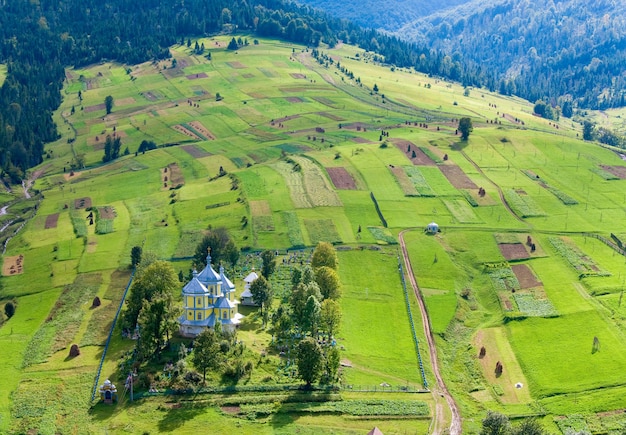This stunning aerial photograph captures a lush, rolling green hill enveloped by tree-covered elevations. At the center of this idyllic scene stands a unique and eye-catching Victorian-style house, characterized by its vibrant blue exterior and four tall, imposing towers. The body of the house is painted a bright yellow, and its windows feature elegant archways, adding to the architectural charm. Nestled behind and to the right of the house, a quaint white gazebo peeks through the dense foliage. The house is cocooned by a multitude of trees, enhancing its secluded and serene atmosphere. The image is devoid of any human presence, animals, or text, allowing the viewer to fully immerse in the tranquility and beauty of the landscape.